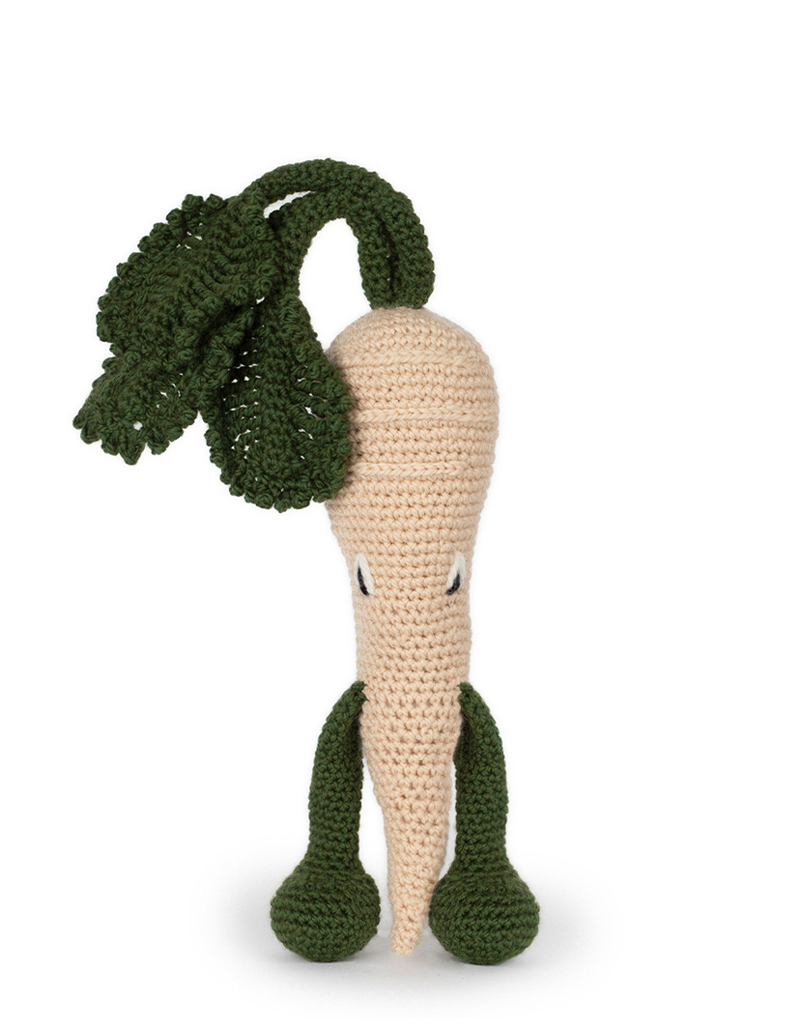This image features a crocheted stuffed toy resembling a root vegetable, possibly a carrot or turnip. The figure is crafted from yarn and displays a beige, tapered body with a pointed bottom and a rounded top that widens. At the top of the head, green stems and leaves sprout outward, while similar green root-like structures are present at the bottom. Notably, the toy has black crochet eyes situated midway up its body, giving it a playful, child-friendly appearance. The entire scene is set against a white background, highlighting the intricate woven details and the vibrant colors of the crochet work.